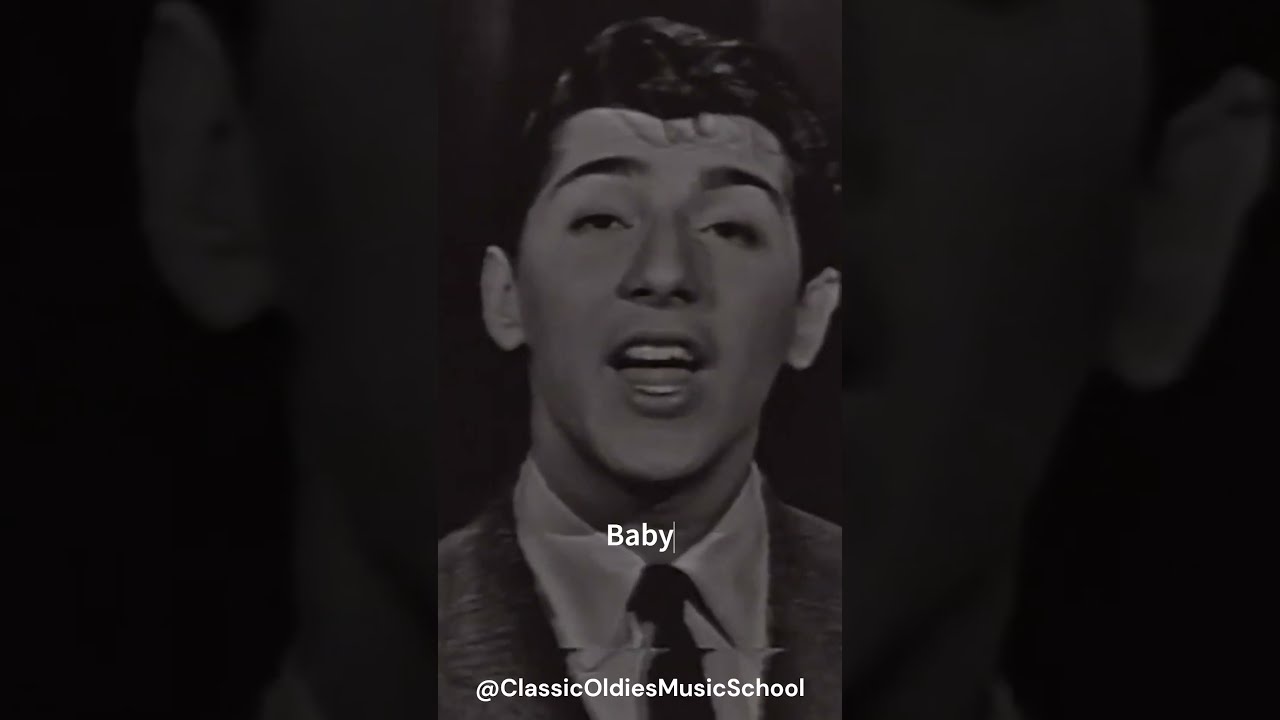In this black and white photograph, we see a close-up of a young Caucasian man, likely in his twenties, with his mouth open as though he’s singing, displaying his teeth. His short hair, greased back or parted to the side, highlights his dark eyebrows. He’s dressed in a dark suit coat, a white button-down shirt, and a black tie. The primary image prominently displays his face and upper chest, while the background features a blurred, darker zoom-in of the outer edges of his face and ears, merged into the overall composition. Overlaid in white text above his tie is the word "Baby," with a cursor seen after the Y, and at the bottom of the image, it says "At Classic Oldies Music School." The photograph evokes a nostalgic, 1950s aesthetic suggested by his attire and style.